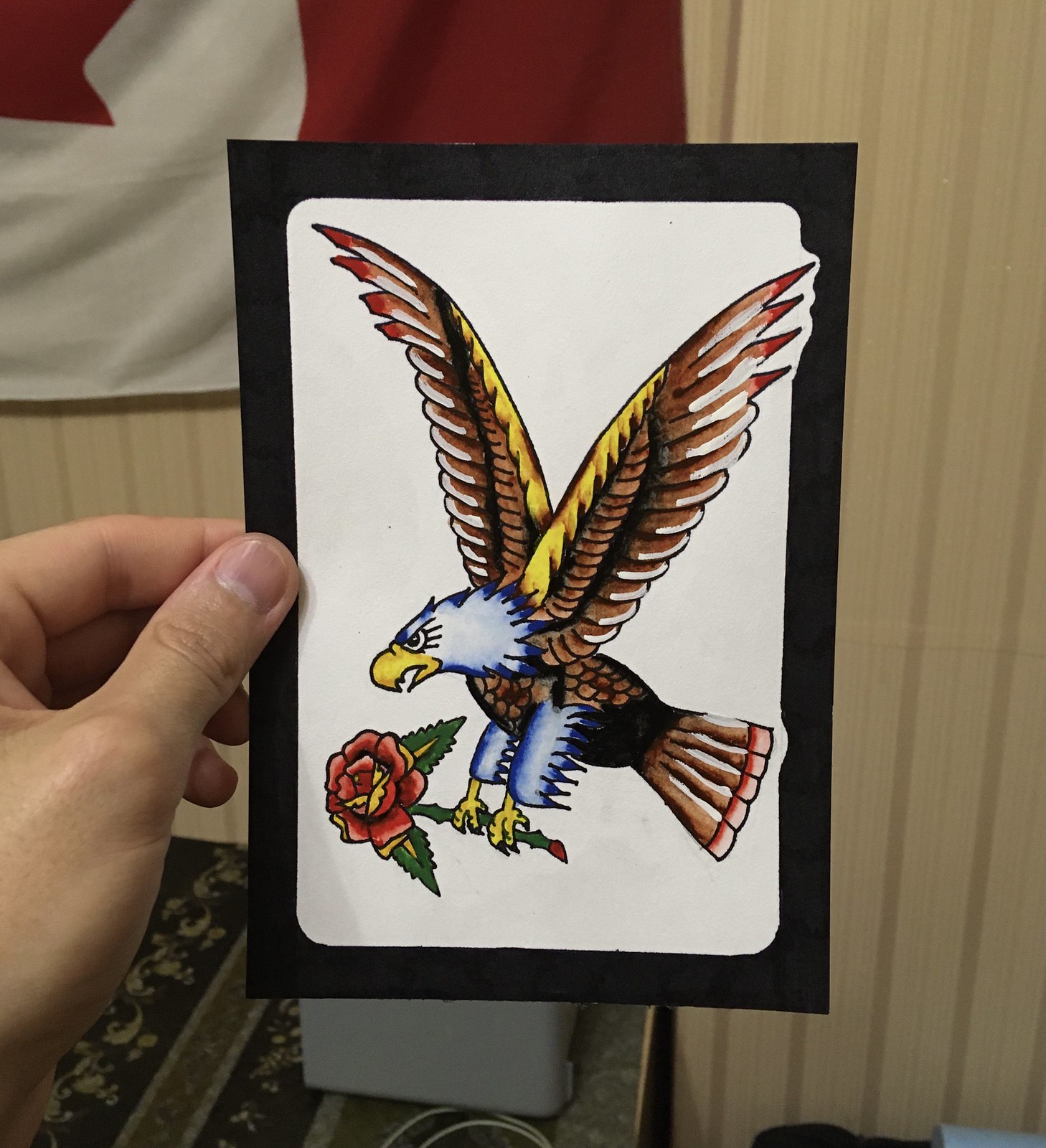In this photograph taken indoors, a person is holding up a black card featuring a central white area bordered in black. Within the white space, an intricately drawn eagle is depicted mid-flight, soaring toward the left. The eagle has a striking white head and legs, complemented by brown wings tinged with shades of yellow, a brown body, and a brown tail. Clutched in the eagle's hanging claws is a single red rose with a vibrant green stem, creating a vivid contrast against the black card.